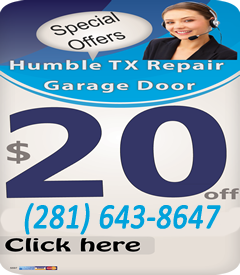This image is a cropped, zoomed-in, and low-resolution snippet of an older advertisement banner for a garage door repair service. The banner features a primary color scheme of blue at the top and off-white for the bottom two-thirds. Prominent dark blue text advertises "$20" followed by light gray text "off". Below this, a contact number "281-643-8647" is displayed in light blue text.

Further down, the words "click here" appear in black text in a different font, positioned above a row of small icons representing various credit cards. At the top of the banner is an image of a woman with light skin, blue eyes, and a smile, wearing a professional power suit with a deep V-neck. She is equipped with a headset, looking directly at the viewer.

Next to the woman, there is a white word balloon with black text that reads "special offers" in a different font. Beneath this, white text states "humble TX repair garage door," indicating the location and nature of the service. The entire image is oddly cropped into a square with cut-off corners, and its poor resolution suggests it might be a blown-up version of a smaller or older internet advertisement.